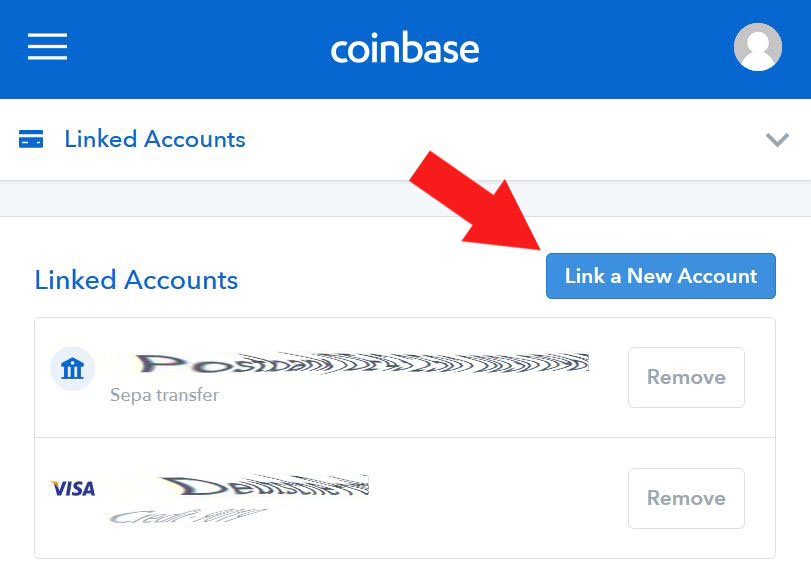The image features a detailed screenshot from the Coinbase app interface, prominently zoomed in to highlight specific elements. The upper portion of the image has a blue background, showcasing the Coinbase logo in white text centered in the top section. To the left of the logo are three horizontal white lines, commonly indicating a menu, while to the right is a profile picture icon set against a grey background.

Below this header, a section with a white background displays the text "Linked accounts" accompanied by a blue credit card icon on the left and a small grey arrow on the right. Beneath this section is another background in grey.

A large red arrow points diagonally downward to the right, drawing attention to a blue button that says "Link a new account" in white writing. To the left of this button, the text "Linked accounts" reappears in blue writing.

Continuing downwards, the user’s first name starts with "P.O" before fading away to the right. Next to the name, it says "SEPA transfer" followed by an outlined "remove" button on the right. Below this entry, the name of a VISA account begins with "D" and similarly fades away. To the right of this entry is another "remove" button.

The entirety of the lower section maintains a white background, ensuring the text and elements stand out clearly. This thorough description encapsulates all elements present in the image, providing a clear and detailed understanding of the Coinbase app interface depicted.